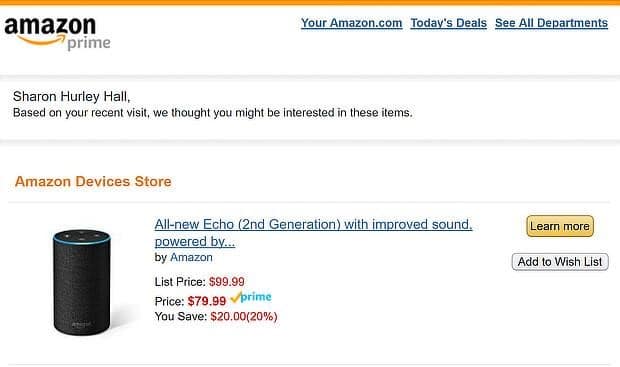Screenshot of an Amazon Prime Shopping Cart:

At the very top of the screenshot is a long, orange bar stretching across the entire width of the image. Directly beneath this bar, on the left-hand side, the word "Amazon" is displayed, followed by "Prime" written in gray. An iconic Amazon arrow graphic, extending from 'A' to 'Z', is nestled near these words. To the right are blue hyperlinks reading "YourAmazon.com," "Today's Deals," and "See All Departments."

Below this section, a black text header states: "Sharon Hurley Hall, based on your recent visit, we thought you might be interested in these items." Directly beneath this is an orange header titled "Amazon Devices Store."

Occupying the left side under the Amazon Devices Store text is an image of an Amazon Echo device, resembling a cylindrical speaker with a blue light ring at its top. Adjacent to the Echo image, a hyperlink text reads: "All-new Echo (2nd Generation) with improved sound, powered by Alexa." Directly below this description is a blue hyperlink that reads "Buy Amazon." 

Further down, the text "List Price" appears, followed by "$99.99" in red. Right below, it states "Price" with a subsequent red price tag of "$79.99." Next to this pricing information, a "Prime" icon is displayed featuring a blue checkmark in front of the word "Prime" in blue, accentuated by an orange background. Below this icon, the savings are highlighted in red text indicating, "You save $20 (20%)."

To the right of the pricing details, a prominent golden button reads "Learn more" in black text, followed by a smaller gray button underneath, labeled "Add to Wishlist" in black text.